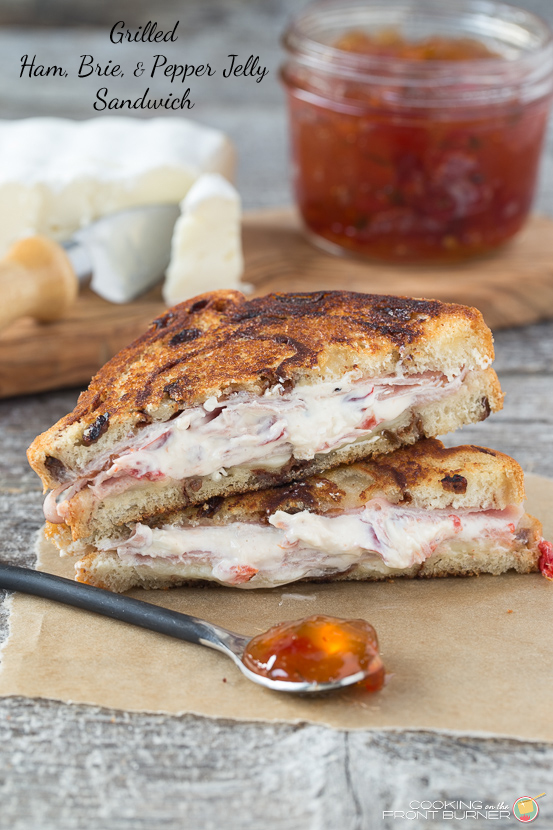This detailed photograph, likely from a recipe blog, features a grilled ham, brie, and pepper jelly sandwich as its focal point. The sandwich is made with swirled cinnamon raisin bread, toasted to a perfect golden brown. It is cut diagonally, with the two triangular halves stacked, revealing the melty brie and flecked pepper jelly spilling out, creating a tantalizing, creamy blend of white and pink at the center. The sandwich is placed on a piece of tan parchment paper, which also holds a small metal spoon laden with amber pepper jelly, the light catching the jelly to give it a golden hue. In the background, on a wooden cheese board, sits a wheel of brie accompanied by a cheese knife, and a ball jar filled with homemade, reddish-brown pepper jelly. The top left corner of the image features the title "Grilled Ham Brie Pepper Jelly Sandwich," and there is a watermark in the bottom right corner, suggesting the picture is from an online recipe site.